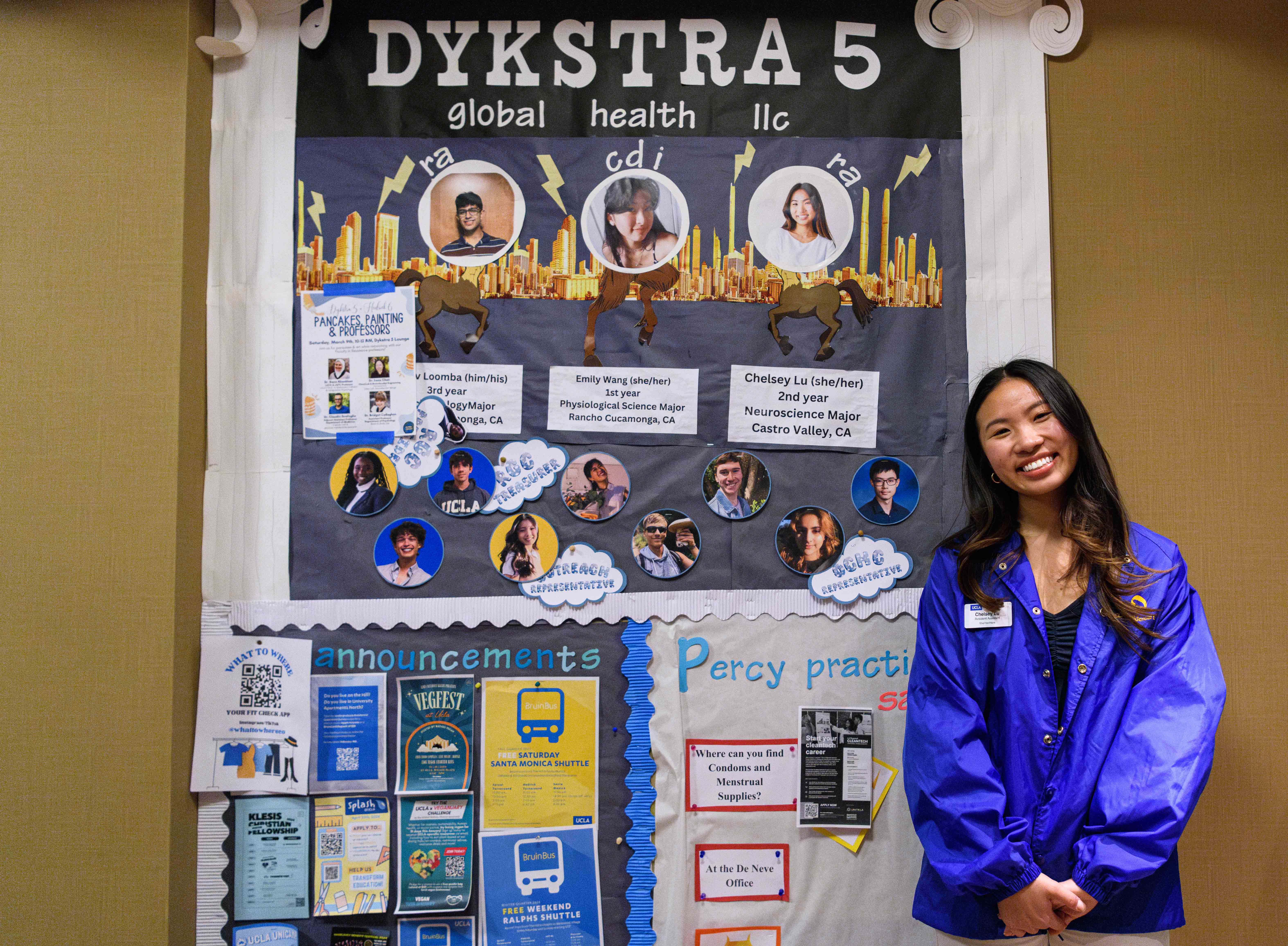The photograph features an Asian woman standing indoors, smiling at the camera with her teeth visible. She is dressed in a blue jacket, which has a name tag pinned to it, a black shirt underneath, and white pants. Her hair falls past her shoulders. Behind her, there is a brown wall with a large, white-framed poster featuring numerous pictures and text. At the top of the poster, "Dijkstra 5, Global Health, LLC" is written. The poster contains circular pictures of people, announcements, and various informational papers. The woman is positioned in front of the poster, which adds a professional and organized context to her cheerful demeanor.